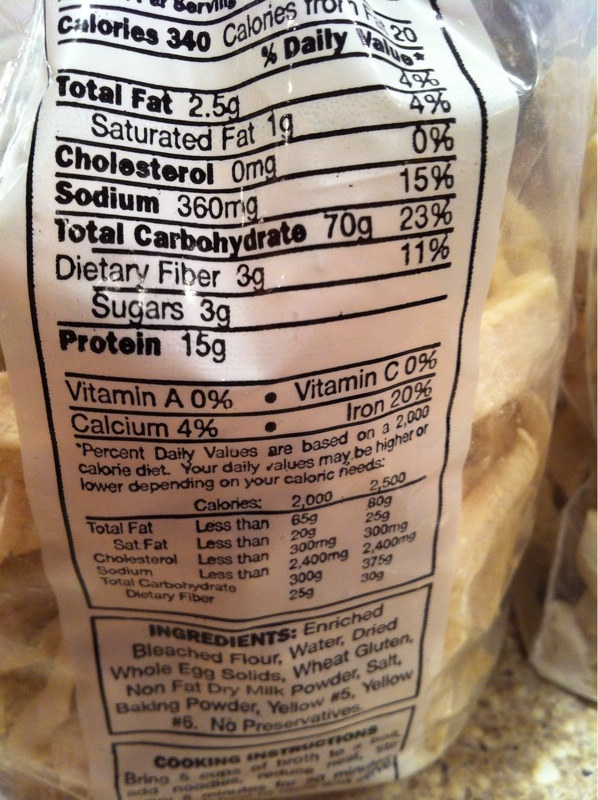This is an up-close photograph displaying the Nutrition Facts label on a clear plastic bag, possibly containing egg noodles or dried pasta. The white rectangular label with black text presents detailed nutritional information: 340 calories, 2.5 grams of total fat, 1 gram of saturated fat, 0 milligrams of cholesterol, 360 milligrams of sodium, 70 grams of total carbohydrates, 3 grams of dietary fiber, 3 grams of sugars, and 15 grams of protein. The label also states the micronutrient content: no vitamin A or vitamin C, 4% calcium, and 20% iron. The ingredients listed include enriched bleached flour, water, dried whole egg solids, wheat gluten, nonfat dry milk powder, salt, baking powder, yellow number five, and yellow number six, with no preservatives. Additionally, the label mentions cooking instructions to bring five cups of broth to a boil, add noodles, reduce heat, with the rest of the instructions blurred.